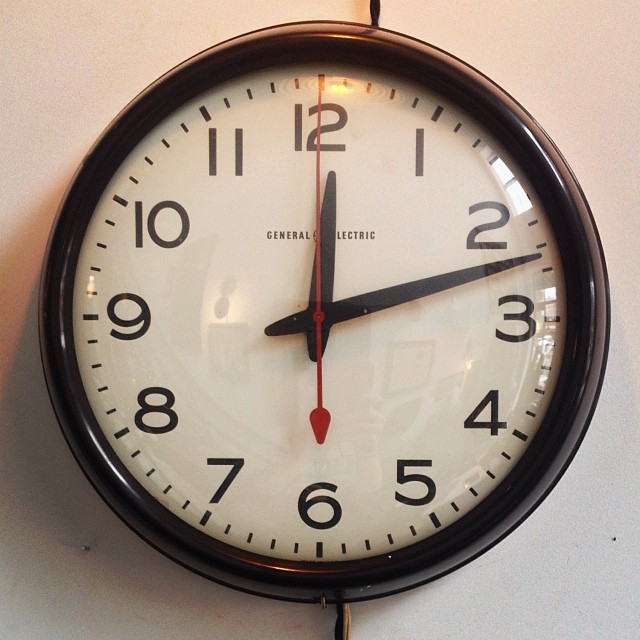This is a photograph of a round, black-rimmed plastic clock set against a slightly dingy white wall with a few nail holes. The clock face has a white background with black numerals arranged counterclockwise. The hour and minute hands are black, while the second hand is red. "General Electric" is written in black text at the center of the clock. The hour hand points at 4, the minute hand just after 2, and the red second hand points at 6. Additionally, the clock has a black string at the top and two strings at the bottom, one black and one light brown. The reflection in the clock reveals a person holding a cell phone to capture the photo, suggesting it was taken indoors, possibly in someone's living room with windows visible off to the right.